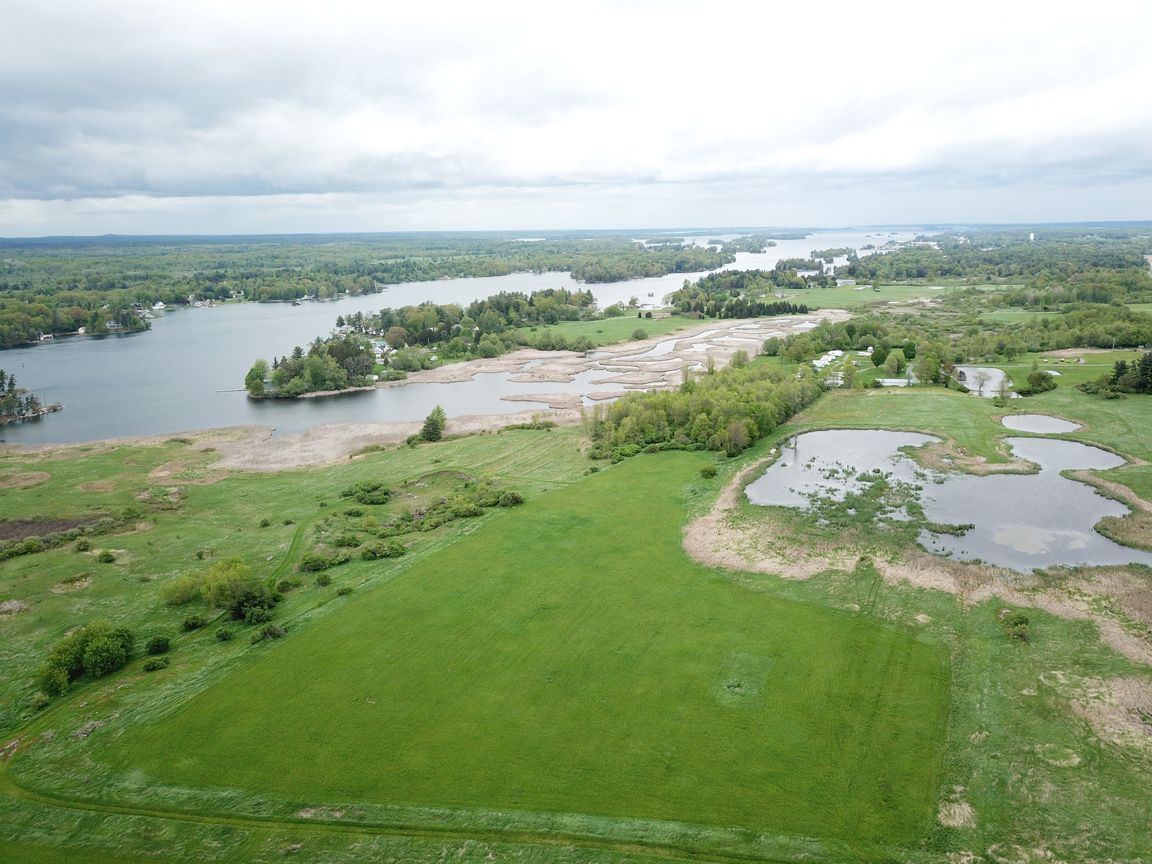This detailed aerial photograph captures a lush wetlands landscape likely taken from a drone, offering a comprehensive view of the area. The foreground showcases a vibrant mix of green fields and dense forestry dotted with shrubs and deciduous trees, suggesting a spring or summer setting. Multiple water bodies are scattered throughout the image, including a substantial river meandering from the left to the center and continuing towards the right. To the right, a noticeable pond with clear water and a brown, rocky shoreline can be seen. The wetlands are marked by numerous small islands and inlets of trees, creating a mosaic of water and greenery. The background features a range of dark hills and distant tree lines, punctuated by a few indistinct buildings, possibly houses. Above, the sky is filled with a mix of white, gray, and blue clouds, hinting at potential rain later in the day. The expansive view encapsulates the serene and untouched beauty of this diverse ecosystem, with no apparent presence of people or animals.